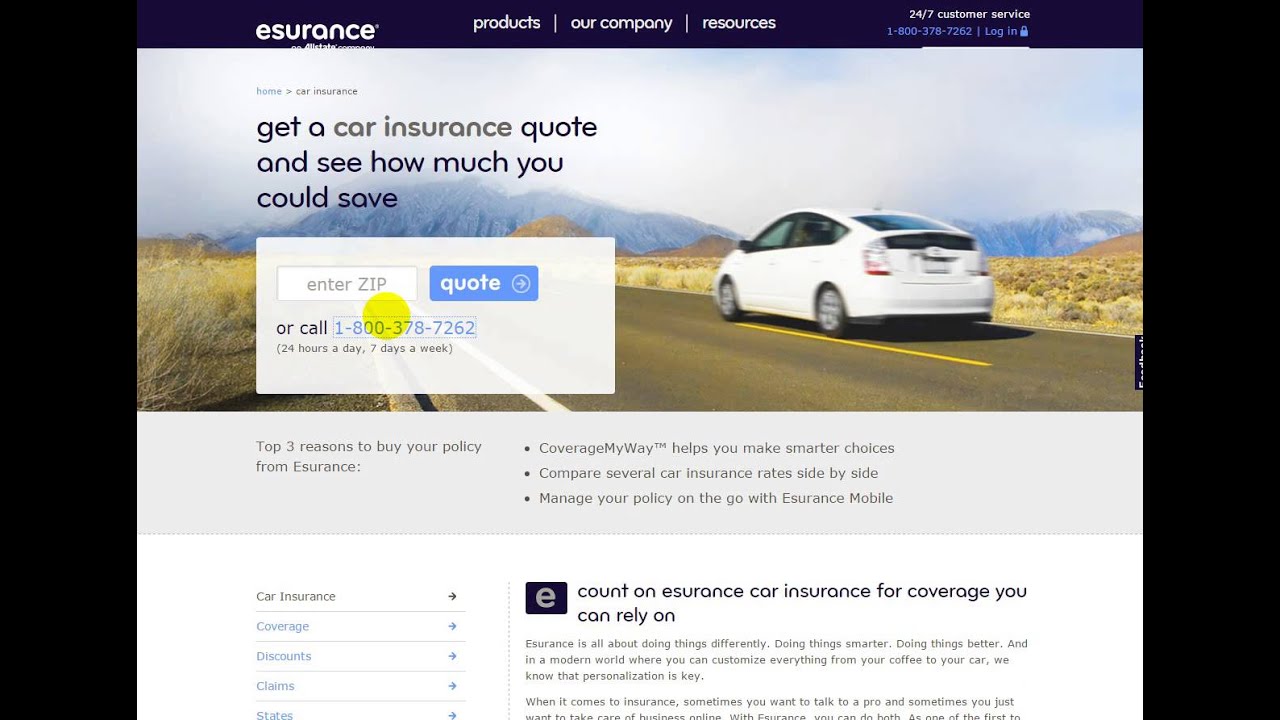In this screenshot, we see the landing page of a website called eAssurance. The background features an image of a person driving what appears to be a Ford Prius, conveying a sense of motion and freedom. The overall color scheme includes a deep navy blue outer layer that frames the page.

At the center of the landing page is a prominent feature—a picture alongside an opt-in form designed for users to get a car insurance quote. This form is accompanied by a pop-up box with a call-to-action that reads, "Get a car insurance quote and see how much you could save or call the number." A yellow circle highlights this message, emphasizing its importance and availability 24 hours a day, 7 days a week.

Above this section, the navigation bar includes links to Products, Company, and Resources, providing easy access to various parts of the website. 

Below the opt-in form is a gray section listing "Three Reasons to Buy Your Policy from eAssurance," providing compelling arguments for prospective customers. Finally, further down, there is a navigational section titled "What to Expect" and a descriptive paragraph outlining the company's strengths and advantages, serving as a persuasive summary of why eAssurance is a great choice for car insurance.